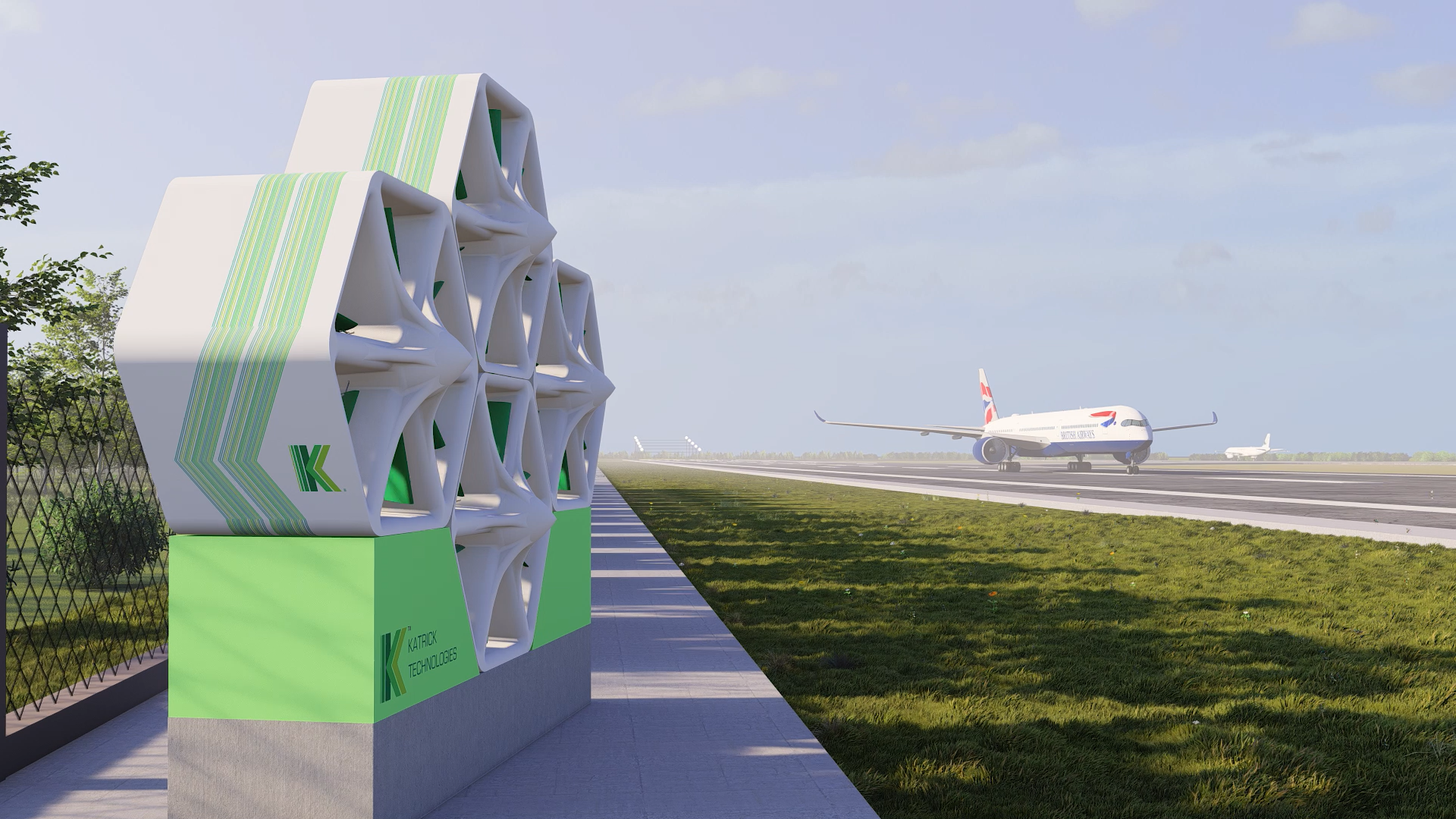This scene captures a commercial jet airliner either taking off or landing on a gray runway, flanked on one side by short green grass. The airliner, a large passenger plane, is predominantly white with a distinctive blue underbelly and engines. Its nose features a striking pattern: a red stripe beginning at the cockpit and curving around to meet the blue. The tail of the plane mirrors this color scheme with two red stripes flanking a central blue stripe, contributing to a visually cohesive design. On the left side of the image, a unique sculpture advertising the airport stands out. It's a white honeycomb-like structure branded with "Catrick Technologies" and adorned with a dark green 'K' logo that transitions to light green where it intersects the vertical element. Nestled between the runway and the sculpture, there is a stretch of maintained green grass, backed by a chain-link fence with trees in the distance. Above, the sky is predominantly blue with a scattering of light gray clouds.